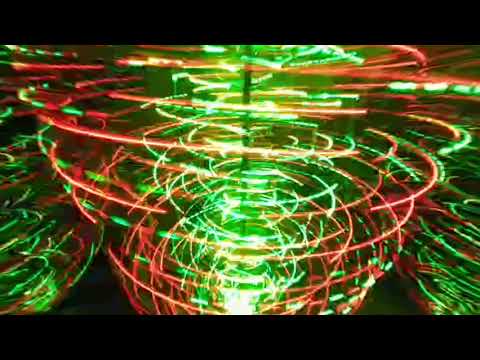The digital art image features three conical vortexes of swirling neon lights, vividly combining green and red hues. The central vortex is fully visible, while the ones on the left and right are partially visible, showing only their edges. Each vortex starts larger at the top and narrows downwards, emphasizing their conical shape. The inner regions of the vortexes glow brightly in green, transitioning to red on the outer edges with occasional specks of yellow. At the top and bottom of the image, there are two plain horizontal black strips acting as borders, framing the vivid neon display.